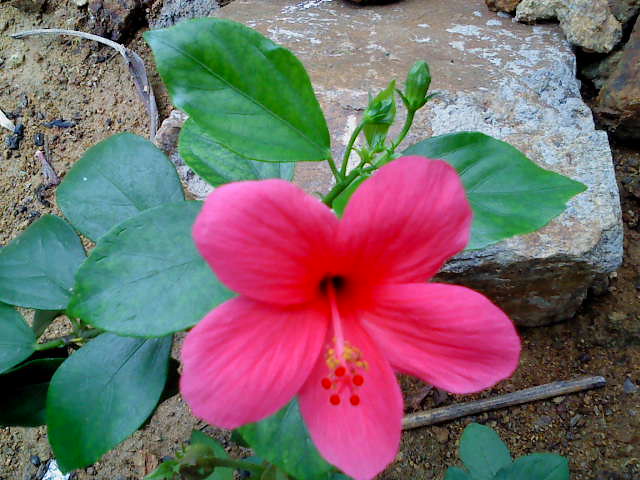This is an outdoor photograph taken on a sunny day, showcasing a tall pink flower, likely a hibiscus, set against a backdrop of coarse, rocky, and slightly damp ground. The rectangular photograph measures approximately four inches tall and six inches wide. The flower, which sits in the middle and extends down to the bottom of the image, features five soft, translucent pink petals that gradient from dark pink at the center to light pink at the edges. A singular long stamen with vibrant yellow and red puffball-like pollen areas protrudes from its center. Green, elliptic-shaped leaves surround the flower, while two closed green buds extend upwards. In the surrounding environment, the ground appears wet and sandy with a collection of small rocks and a large square stone located in the upper right corner. Additional details include a small stick and three green leaves from another plant at the base of the flower, along with a piece of flat slate rock and brown dirt, creating a rich, textured background highlighting the delicate beauty of the hibiscus flower.